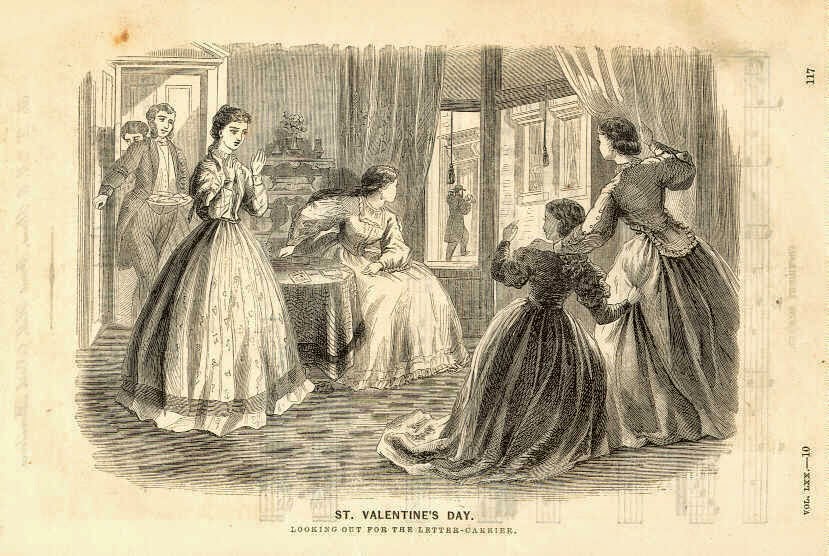This image features an intricately detailed, old-fashioned drawing—possibly taken from an antique book—characterized by its slightly yellowed, orange-tinted, and lightly stained paper. The black-and-white illustration depicts a domestic scene set in a parlor, showcasing men and women in elaborate, Victorian-era attire, typified by their puffy sleeves, long poofy dresses, and petticoats. On the far left, a woman with dark hair and a floral patterned dress stands near a door, seemingly about to applaud. To her right, another woman is seated at a desk, her head turned towards the window, as if distracted by the activities outside. 

In the center of the image, two women (or a woman and a girl) are seen standing by a window, holding the curtain open and peering out with surprised expressions. Outside the window, a man appears to be knocking on a door across the street. Simultaneously, an entrance scene unfolds on the left side of the illustration where two gentlemen are entering the room—one is seen opening the door while holding a platter of food, and another person's head is just visible behind him. The image's vintage feel is underscored by a caption beneath it reading, "St. Valentine's Day," followed by additional, smaller text that is too faded to decipher.